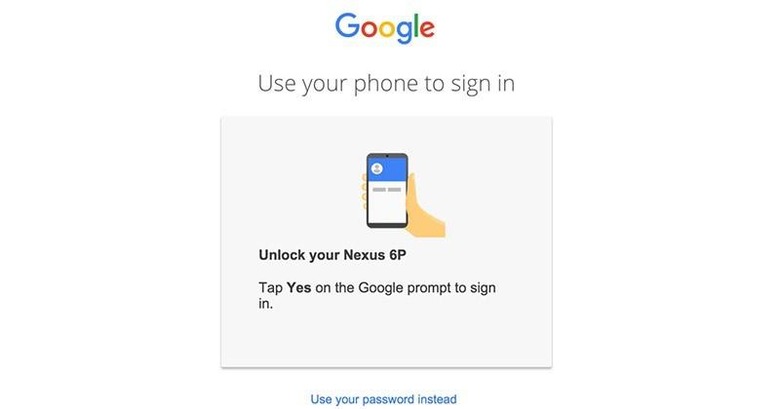The image displays a set of instructions for signing into a Google account using a Nexus 6P smartphone, set against a white background. 

At the top of the image, the Google logo is prominently featured. Below the logo, it reads, "Use your phone to sign in." 

Directly under this text is a rectangular box shaded in a slightly darker tone of white. Within this box, there is an illustration of a hand holding a smartphone. Beneath this illustration, two lines of black text provide further instructions: "Unlock your Nexus 6P" and "Tap Yes on the Google prompt to sign in."

Below the rectangular box and back against the brighter white background, there is a clickable link that says, "Use your password instead."

This image serves as a step-by-step guide for setting up a Google account on a Nexus 6P smartphone, offering the option to either use a Google prompt or an account password for the sign-in process.